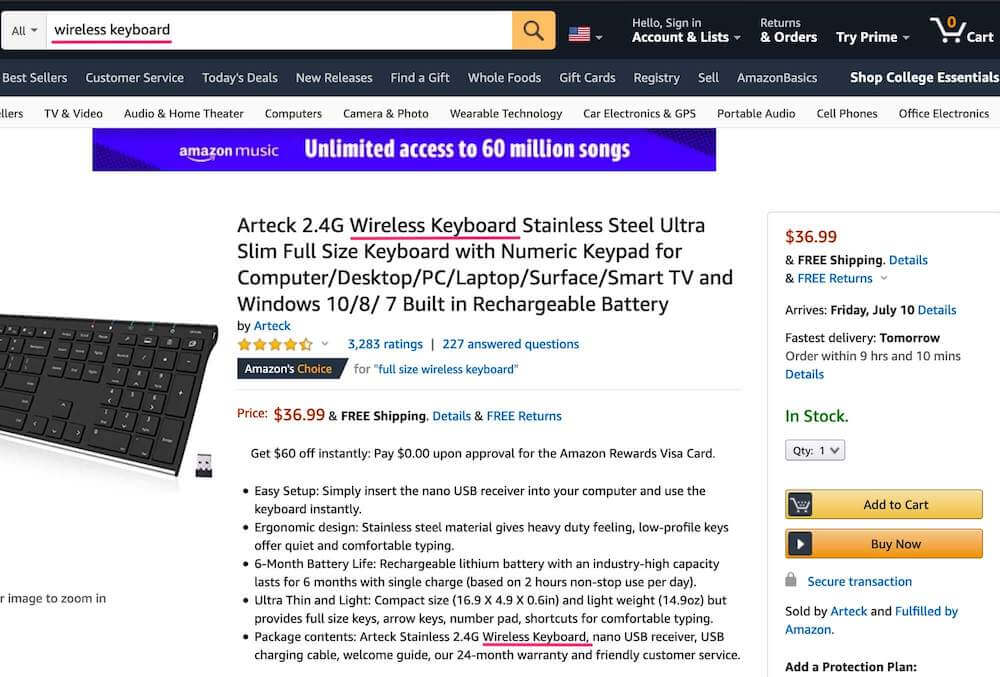An Amazon webpage is displayed, detailing a search for a "wireless keyboard." At the top left, a dropdown menu labeled "All" appears next to the search bar where "wireless keyboard" has been entered. An orange magnifying glass icon accompanies this search bar. The page is set to the U.S. region, indicated by the American flag, allowing users to switch their shopping region.

To the right of the search bar, navigation options include "Hello, Sign in Account & Lists," "Returns & Orders," and a prompt to "Try Prime." The cart currently shows zero items. Beneath this navigation bar, quick links to "Best Sellers," "Customer Service," and "Today's Deals" are visible.

The subsequent row mirrors the previous links but adds categories such as "TV and Video" and "Audio," although this section is partially cut off. A prominent blue banner advertises Amazon Music, boasting access to 60 million songs.

Highlighted below the banner is an advertisement for an Air Tech 2.4G Wireless Keyboard. The ad describes it as a stainless steel, ultra-slim, full-size keyboard, featuring a star rating system. The price of the keyboard is listed at $36.99, including free shipping. Bullet points provide further details, and a promotion promises an instant $60 off with the use of an Amazon Rewards Visa card.

To the left of the advertisement, a partial image of the keyboard is displayed. On the right, a boxed section reiterates the price and free shipping offer, confirming the item is in stock. It also indicates an estimated delivery date of July 10th. Below that are yellow buttons for "Add to Cart" and "Buy Now," facilitating immediate purchase options.